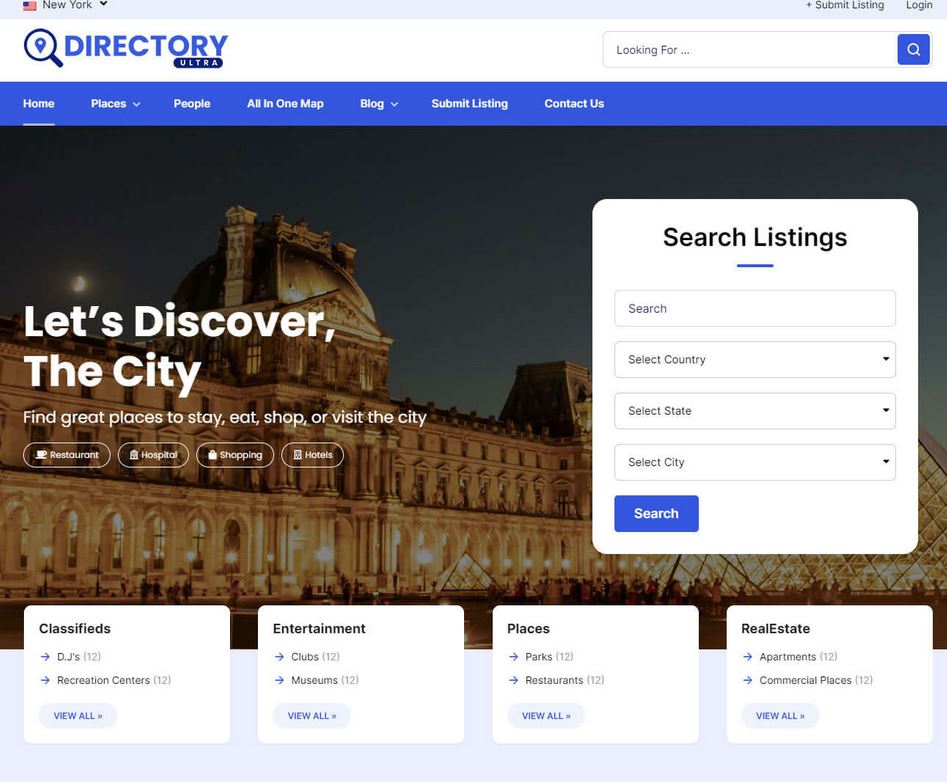Screenshot of Directory Ultra's Homepage

The screenshot showcases the homepage of the website called Directory Ultra, which features a clean and user-friendly design. At the top left, the website's logo is prominently displayed in large, bold blue letters. To the right, a large search box occupies a significant portion of the page, with the phrase "looking for" in small black letters inside the box and a blue magnifying glass icon for initiating the search.

Immediately below the logo and search box, there is a navigation banner with several options: Home, Places, People, All in One Map, Blog, Submit Listing, and Contact Us. The 'Home' option is currently selected, indicated by a small white line underneath it.

The main visual element of the page is a background photograph of the Louvre. On the left side of this image, large white text overlays reading "Let's discover the city," complemented by smaller white text below it stating, "Find great places to stay, eat, shop, or visit the city." Beneath this text are four buttons labeled Restaurant, Hospital, Shopping, and Hotels, positioned to guide users towards various categories.

On the right side of the background image, there's a large white box titled "Search Listings" in bold black letters. This box features several input fields including a text box for general search, a dropdown menu for selecting a country, another for selecting a state, and a third for selecting a city. A blue 'Search' button is located on the bottom right of this white box.

At the very bottom of the page, there are five horizontally aligned white boxes, each representing different categories with associated subcategories and their respective counts in parentheses:
1. Classifieds: DJs (number of DJs) and Recreation Centers (number of recreation centers), with a 'view all' link.
2. Entertainment: Clubs (number of clubs) and Museums (number of museums), including a 'view all' link.
3. Places: Parks (number of parks) and Restaurants (number of restaurants), along with a 'view all' link.
4. Real Estate: Apartments (number of apartments) and Commercial Places (number of commercial listings), also with a 'view all' link.

This detailed layout provides an intuitive navigation experience, enabling users to easily search and explore various listings within the city.